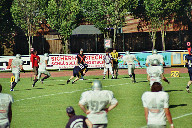The image depicts a closely-contested moment in a football game. One team, dressed in white jerseys with blue numbers, is positioned near the end zone, hinting at a potential scoring opportunity. A player clad in black is shown in a falling motion, possibly holding the ball, adding to the tension of the scene. On the sideline, several players watch intently. The football field is bordered by advertisements, including a blue one, a white one with red lettering, and another in white with black lettering. Adjacent to the field is a brown building adorned with horizontal lines. A referee stands nearby, focused on the unfolding action.